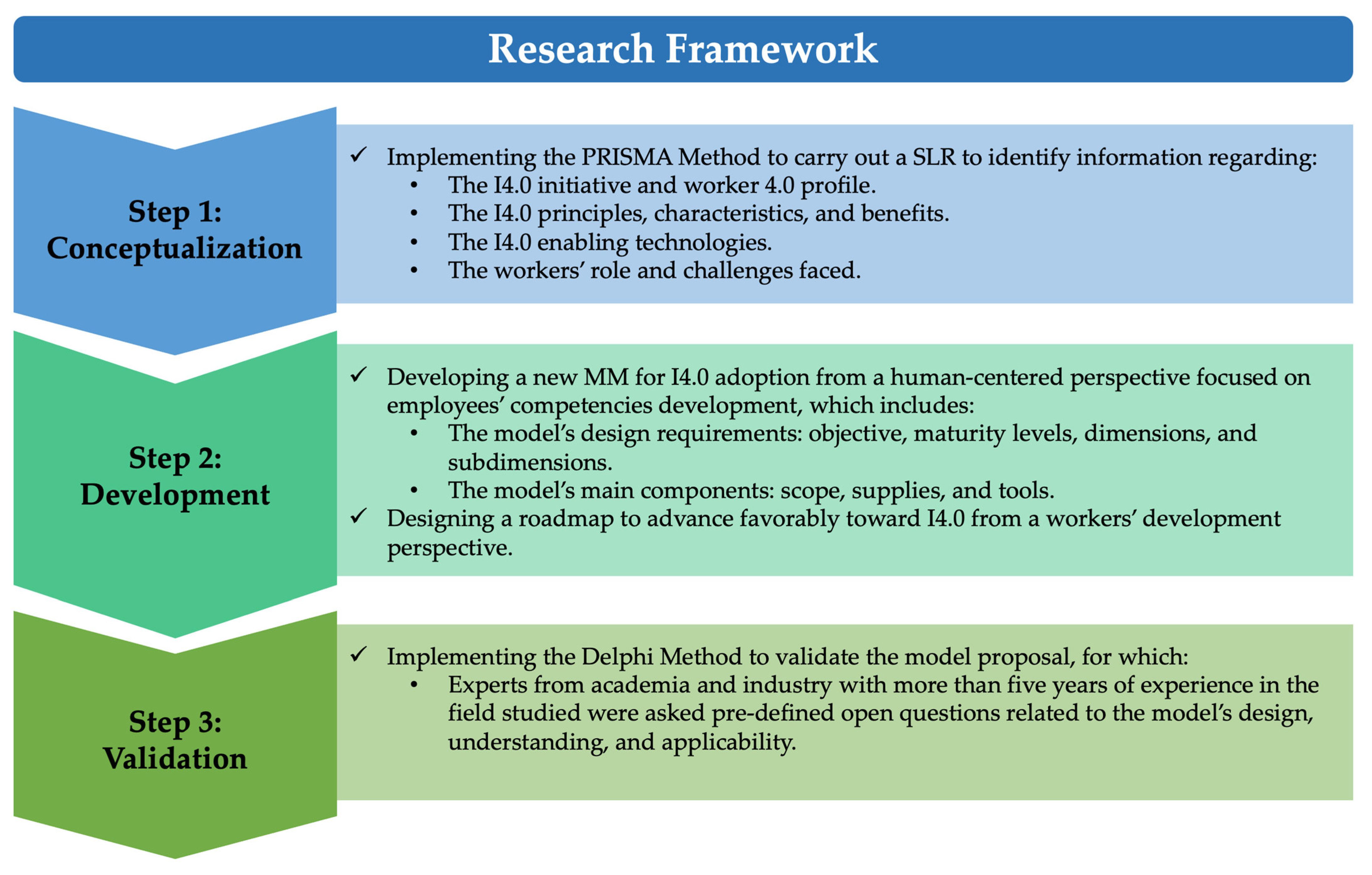The image is a detailed, colorful depiction of a research framework, structured into three main steps: Conceptualization, Development, and Validation. The background features a gradient of blue, light blue, dark blue, light green, and dark green hues. 

On the far left of the image, there are three downward-pointing V-shaped arrows, one placed behind each labeled step. The steps are aligned vertically with "Step 1: Conceptualization," "Step 2: Development," and "Step 3: Validation," each in a visually distinct blue, green, and dark green box, respectively. 

To the right of each labeled arrow, more detailed descriptions are provided in a series of blue, green, and dark green boxes filled with small black text. These boxes include check marks and bullet points summarizing the specific tasks and objectives of each step:

- **Step 1: Conceptualization** involves implementing the PRISMA method to conduct a systematic literature review (SLR) to gather information about the Industry 4.0 (I 4.0) initiative, worker 4.0 profiles, principles, characteristics, benefits, enabling technologies, and worker roles and challenges.
- **Step 2: Development** focuses on creating a new maturity model (MM) for Industry 4.0 adoption from a human-centered perspective, emphasizing employee competency development. It includes designing requirements, objectives, maturity levels, dimensions, sub-dimensions, main components, scope, supplies, and tools, along with a roadmap advancing towards Industry 4.0 from a worker development standpoint.
- **Step 3: Validation** utilizes the Delphi method to validate the proposed model by consulting experts from academia and industry with over five years of experience. These experts are asked predefined open questions to evaluate the model’s design, understanding, and applicability.

Overall, the image seems styled like a page from a textbook or web page, providing a structured and colorful guide to executing a research project using this specific research framework.